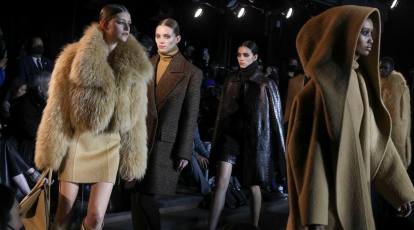The image depicts a vivid fashion event with four striking models showcased against a backdrop featuring an audience and overhead lights, suggesting a runway setting. Starting from the left, the first model is a white woman with dark brown hair, wearing an oversized beige fur coat with a matching skirt and carrying a tan handbag. Beside her, the second model, also white with slicked-back brown hair, dons a sleek brown trench coat over an orange turtleneck. Moving to the right, the third model, with black hair, sports a large black leather coat paired with black tights. The final model on the far right is a black woman wearing an extensive, suede-like coat with a distinctive hood that gives her an enigmatic, Jedi-like appearance.